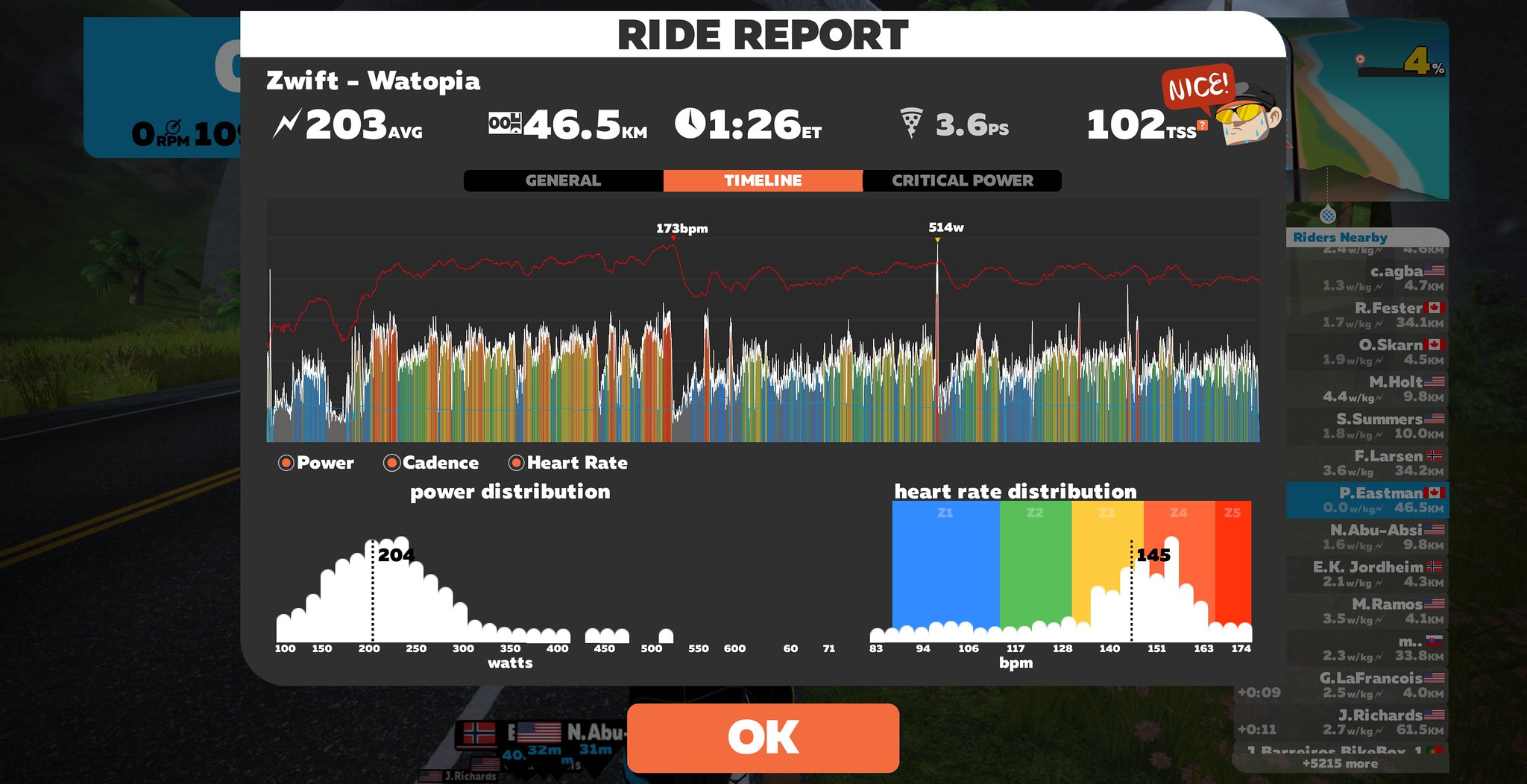The image is a screen capture of a statistics-filled window from what appears to be a riding simulation game named Zwift, set in a place called Watopia. At the top of the window, in a white strip with gray text, it reads "Ride Report." Directly below, it lists several statistics: 203 AVG (average power), 46.5 KM (distance), 126 ET (elapsed time), 3.6 PS (presumably power score), and 102 TSS (training stress score). The interface features three tabs: General, Timeline, and Critical Power, with the Timeline tab highlighted in orange.

Central to the window is a colorful line graph that traces metrics such as power, cadence, and heart rate, characterized by vibrant orange, blue, and yellow lines, with a distinct red squiggly line overlay. Below this, the display shows two bar graphs: one labeled "Power Distribution" featuring watts along the x-axis, and another labeled "Heart Rate Distribution" with BPM (beats per minute) on the x-axis. These graphs use a color scheme of blue, green, yellow, and various shades of orange.

In the lower section of the image, there's an orange rectangle with white text that says "OK." The background of the window suggests a racing game environment, showing a blacktop road and grass on the sides. The overall color palette includes dark gray, black for the background, and white text, which contrasts sharply with the colorful graphs and highlighted sections. An animated graphic of a character giving a thumbs-up with the caption "Nice" adds a bit of visual flair to the analytical display.